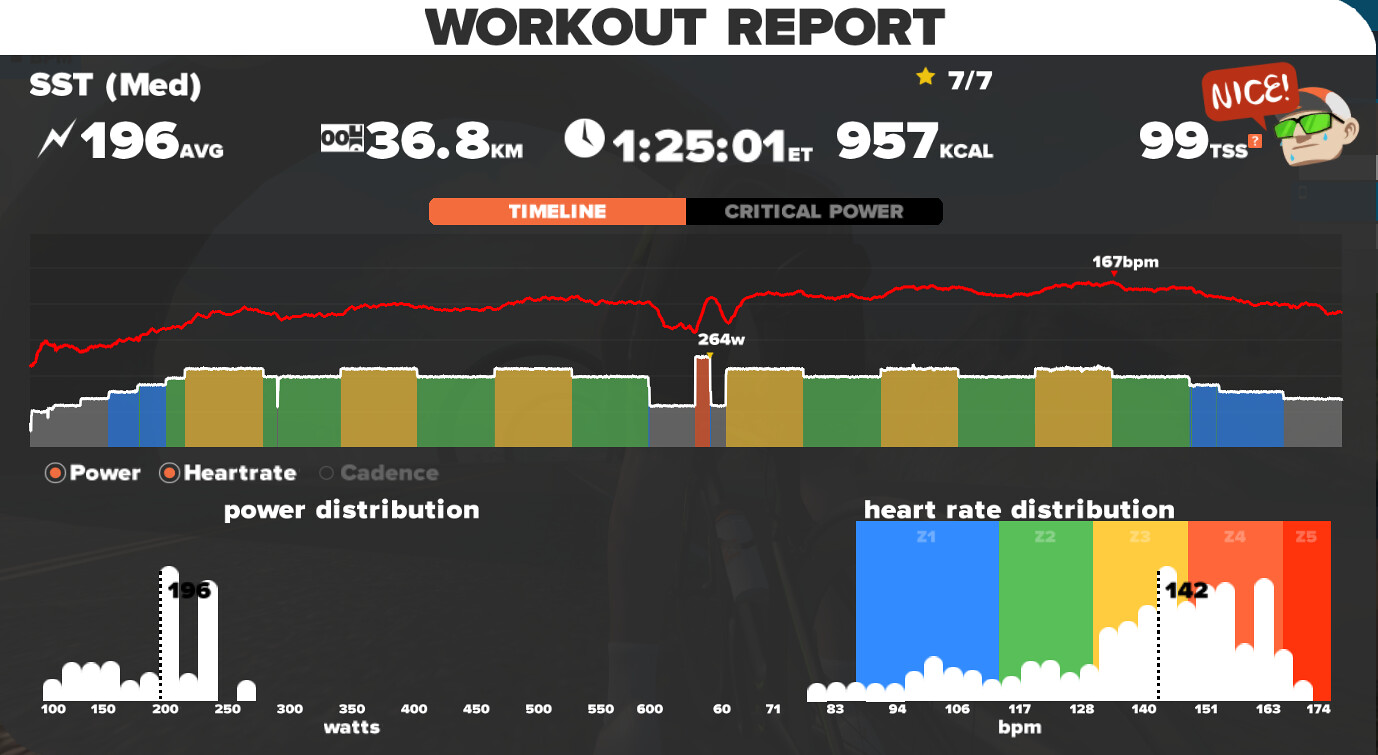The image is a detailed workout report from a health app, showcasing numerous data and statistics on a black background with a colorful interface. At the top, it displays "SST Med" with an average of 196, and reports a total distance of 36.8 kilometers covered in 1 hour, 25 minutes, and 1 second (ET). It also shows 957 kilocalories burned and a Training Stress Score (TSS) of 99. On the right side, there's a cartoon face wearing a hat and green sunglasses, saying "Nice."

Below this section, a timeline features line graphs illustrating power and heart rate metrics throughout the workout, with heart rate data highlighted by a red line. The bottom of the report contains two bar graphs: one on the left for power distribution measured in watts, and one on the right for heart rate distribution, measured in BPM (beats per minute). The colorful graphs incorporate grays, blues, golds, greens, with the heart rate being prominently displayed in red. Additional metrics mentioned include critical power at 264 watts and maximum heart rate at 267 BPM.